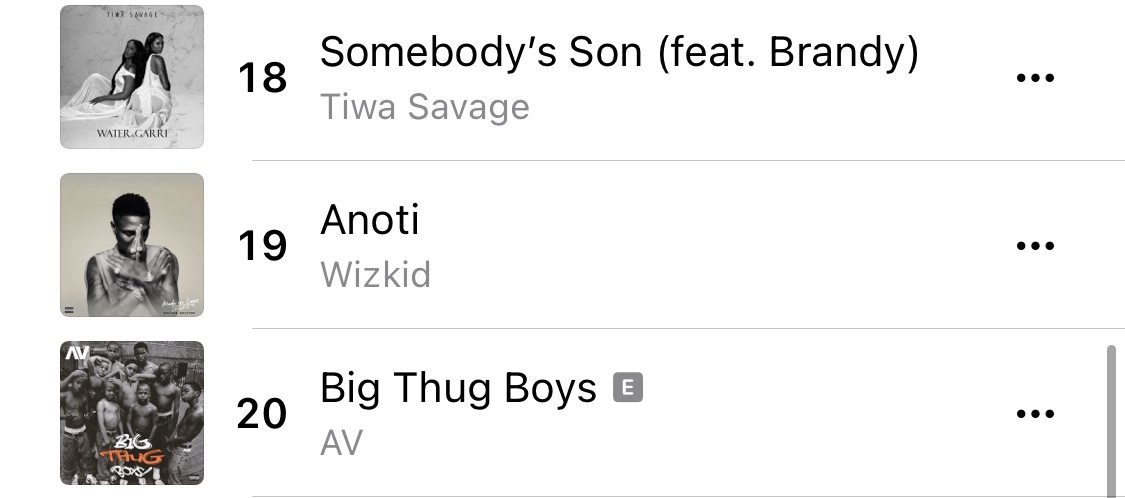Screenshot of a music app (exact app unknown) displaying the bottom three entries of a Top 20 chart. The section shown features entries ranked 18 through 20, each with their accompanying album covers and details:

1. **Number 18:**
   - **Album Cover:** Two African-American women in white dresses sitting back-to-back against a marble background.
   - **Song:** "Somebody's Son" featuring Brandy.
   - **Artist:** Teewa Savage.
   - **Additional Features:** Three dots menu on the right for additional options.

2. **Number 19:**
   - **Album Cover:** An African-American male with short hair, arms crossed over their chest, looking downward.
   - **Song:** "Anoti."
   - **Artist:** Wizkid.
   - **Additional Features:** Three dots menu on the right for additional options.

3. **Number 20:**
   - **Album Cover:** Several young African-American boys, shirtless and in jeans, some making gang signs.
   - **Song:** "Big Thug Boys."
   - **Artist:** A-V.
   - **Symbols:** Letter "E" in a light gray square next to the song title, possibly indicating an explicit content warning.

A scrollbar is on the far right, currently scrolled to the bottom, confirming the visibility of the last three entries on the list.